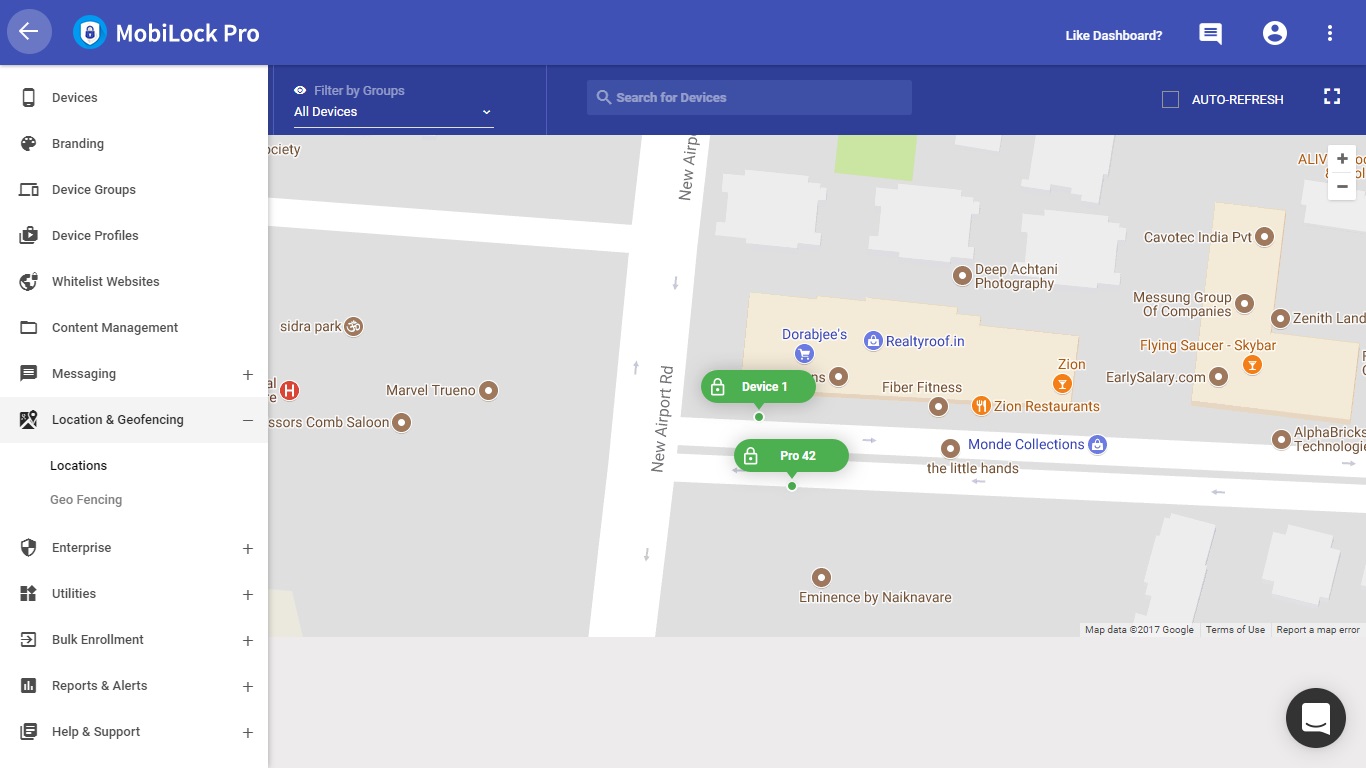The image displays a screenshot of a mobile application named "Mobile Lock Pro." The app’s icon features a blue circle with a white emblem and a blue lock at its center, resembling a coat of arms. 

On the left side, there is a light purple circular icon with a white arrow pointing left. Beneath this, a vertical white section lists various functions organized from top to bottom: Devices, Branding, Device Groups, Device Profiles, Whitelist, Websites, Content Management, Messaging, Location and Geofencing, Enterprise Utilities, Bulk Enrollment, Reports and Alerts, and Help and Support. Each function is accompanied by a distinct icon.

On the right, there is a purple block with an eyeball icon labeled "Filtered by Groups." Below this, a white bar titled "All Devices" (with "A" and "D" capitalized) features a down arrow and a magnifying glass icon, both in grey. To the right of this bar, there is a "Search for Devices" field shaded in purple, next to a white square labeled "AUTO REFRESH" (in all caps). Another fragmented white square has a purple center next to it.

Below these elements, a map displays with streets and a vertical white street marked "New Wear Parrot Row." The streets are bordered by areas shaded in grey and tan, and brown dots marked with letters are scattered across. At the bottom of the map, there is a brown-black circle containing a white piece of paper icon with a downward arrow. A tan area stretches from left to right at the extremes of the map, providing a boundary.

The overall user interface appears to be quite detailed and navigation-focused, highlighting different interactive components for managing devices and their related functions.